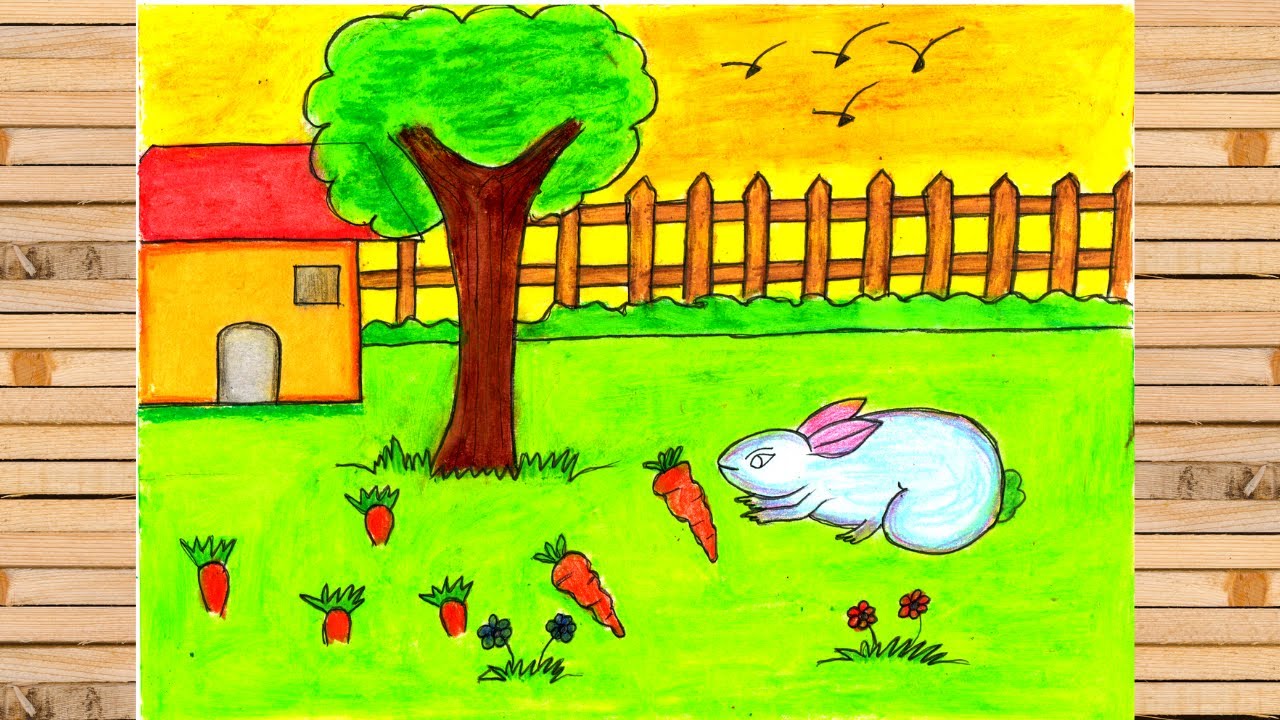This is a detailed drawing, likely done by a child, displayed on a wooden background. The scene depicts a vibrant backyard. At the center of the drawing, there is a prominently featured white rabbit with pink ears and a green tail, fixated on a carrot close to it. Surrounding the rabbit are six carrots: two fully uprooted lying on the lime green grass, and four partially buried in the ground. On the left side of the drawing stands a gigantic tree, next to which is a small house with a red roof, a grey door, and yellow-orange walls. To the right of the house extends a light brown fence, above which four birds are flying. The background of the entire scene, including the grass and other elements, has a whimsical and colorful charm typical of children's artwork.